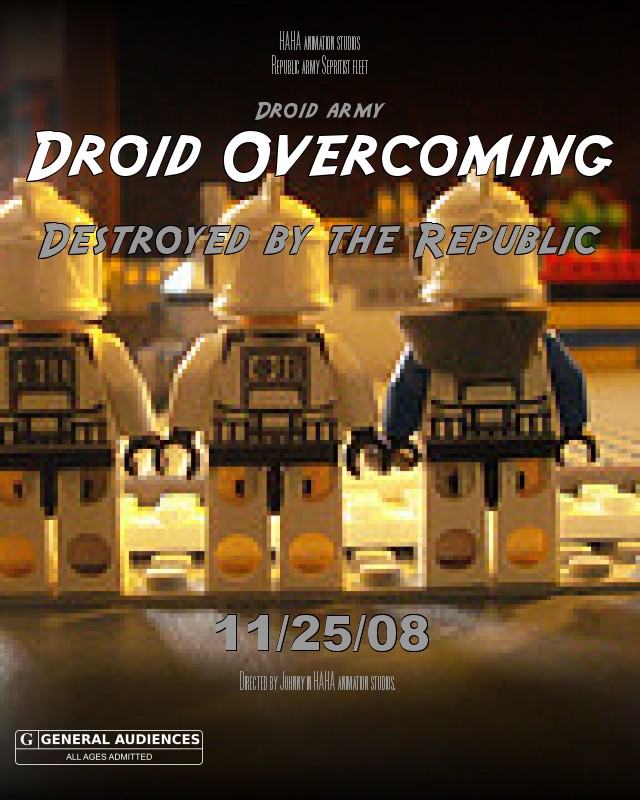The image appears to be an advertisement for a movie or game created by Haha Animation Studios. It prominently features the following text elements: "Haha, Animator Studios," "Republic Army," "Separatist Fleet," "Droid Army," "Droid Overcoming," and "Destroyed by the Republic." The release date is indicated as November 25th, 2008, and it is directed by Johnny. The content is rated G, for General Audiences, allowing all ages to view it.

At the center of the image are three Lego Star Wars figures. The quality of the photo is quite poor, appearing blurry and unprofessional, suggesting that the image might be a humorous or parody advertisement. The Lego figures are arranged with two dressed in all white armor on the left and one in white pants with a blue and white shirt, possibly bearing a hoodie or a bag, on the right. They are set against a Lego backdrop that includes colors like red and green, reminiscent of leaves, and a larger grey Lego structure resembling a chalkboard with black and brown outlines.

The lower portion of the image features the date "11-25-08" alongside credits including "directed by Johnny" and "Haha Animation Studios" in grey letters. In the bottom left corner, the rating "G for General Audiences, All Ages Admitted," is displayed in white letters on a dark background. Overall, the image gives off the impression of an amateurish, perhaps tongue-in-cheek, promotional poster for a fan-made or unofficial Lego Star Wars movie.